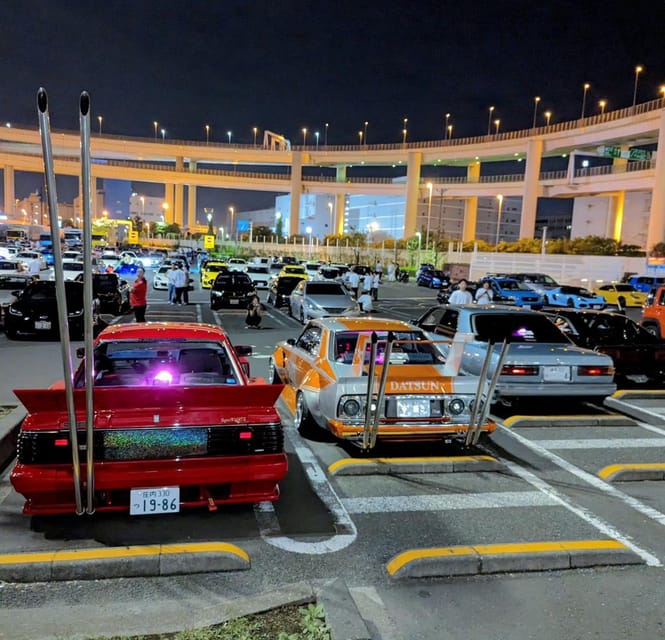In this nighttime photograph, a bustling parking lot stretches beneath a sprawling, multi-tiered highway overpass, bathed in the glow of numerous streetlights. Dominating the foreground is a row of distinct cars, each parked haphazardly; some backed in and others pulled forward. The centerpiece is a striking red sports car adorned with a red fin and bearing the license plate "1986." To its immediate right stands a retro-styled sports car featuring a gray body, prominent orange striping down its center and sides, and an orange sun decal on the back fender. A cyan car and a black car are lined up further to the right. Scattered throughout the scene are numerous individuals, most donning white shirts paired with jeans or black pants. Notably, a man in a red shirt and black pants admires the red car, while a woman, clad in black, crouches beside the orange-striped car, both set against a backdrop peppered with other cars of various hues—black, gray, orange, and white. The landscape hints at an urban Japanese setting, potentially near an airport or concert hall, given the visible Japanese characters on some of the license plates and the extensive highway infrastructure above. The ambiance is vibrant, capturing both the retro charm of the featured cars and the modern hustle and bustle of a metropolitan nighttime scene.